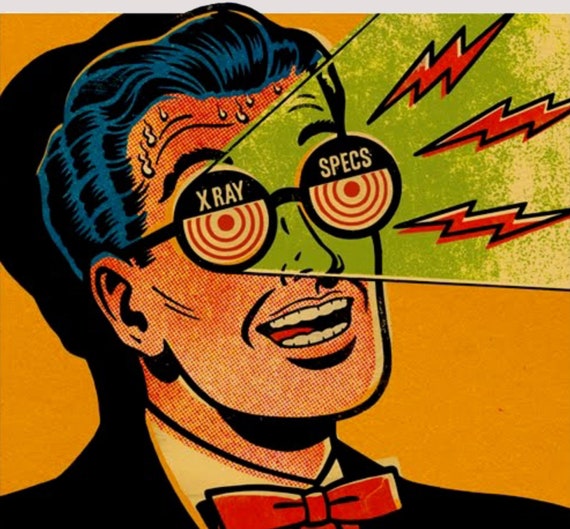The image depicts a cartoonish scene of a sharply dressed young man with bluish-black hair, wearing a black suit, a slightly yellow-toned white button-up shirt, and a reddish-orange bow tie. His mouth is wide open, revealing his teeth and a red tongue, and his forehead shows signs of stress with a reddish tint and white beads of sweat. He’s wearing black glasses with a unique design: the left lens reads "x-ray" while the right lens reads "specs," and both lenses feature a red swirl with a central dot, giving the impression of a hypnotic target. From his mesmerized eyes, a green cone is projected, filled with vivid red lightning bolts, adding to the intense and almost surreal visual effect. The background is predominantly yellow with an orange gradient, and his silhouette is cast dramatically behind him.